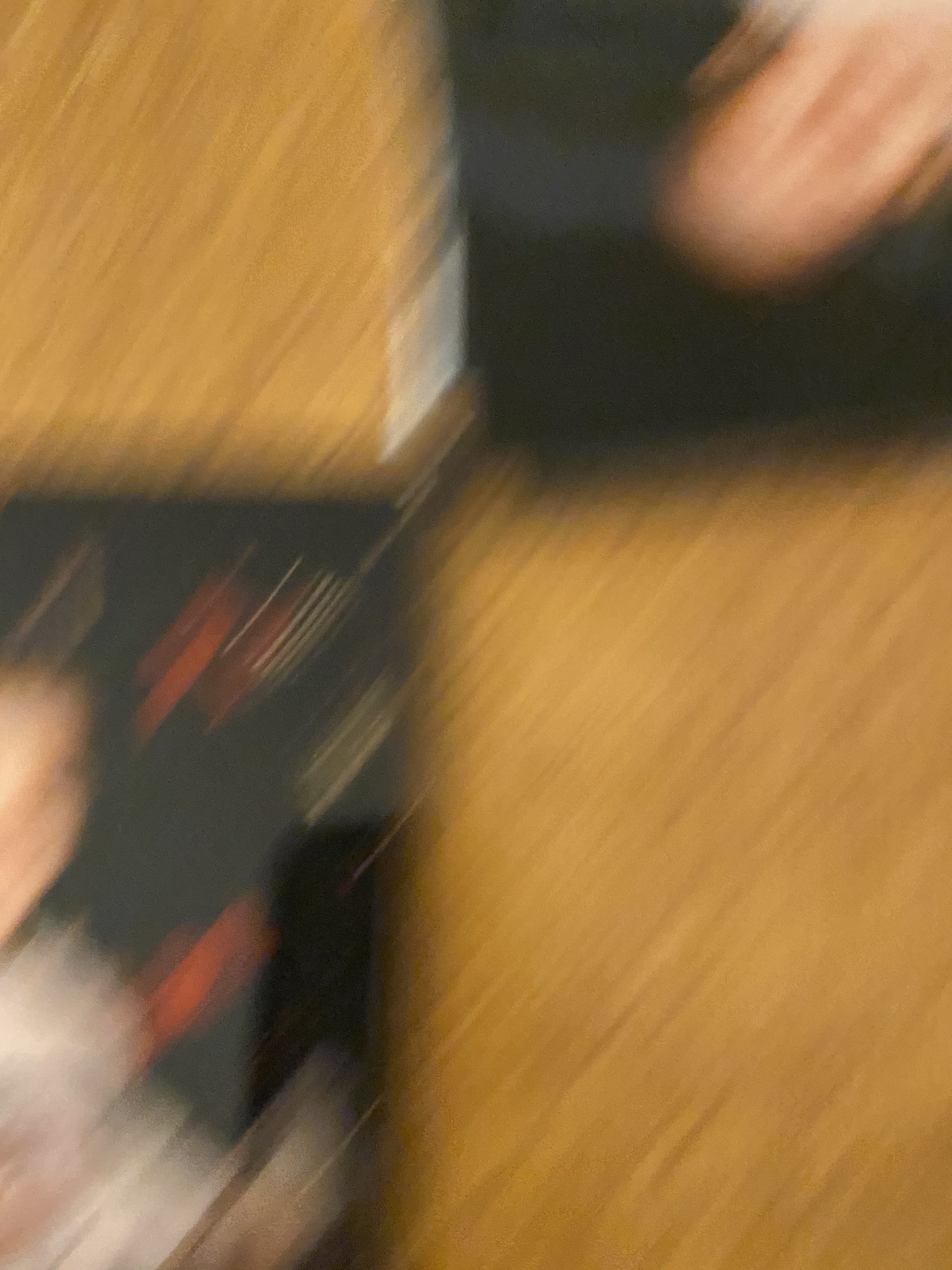In this image, various abstract elements blend into an overall blurred composition. In the upper left corner, a gold-colored box is visible, accented with a white label on its right side. Below this box, there are areas of black interspersed with streaks of gold and orange. Moving to the bottom left, the image features streaks of white and light beige with hints of orange. In the upper right corner, a section of light beige is streaked with brown, all surrounded by a darker brown.

Dominating the middle to the bottom right is another large box, also gold with brown streaks, mirroring the one in the upper left corner. All these elements are set against a dark brown to black background, creating a disjointed and unclear visual that makes it difficult to discern specific objects or details. The overall impression is one of looking at the border of something due to the significant blur obscuring finer details.